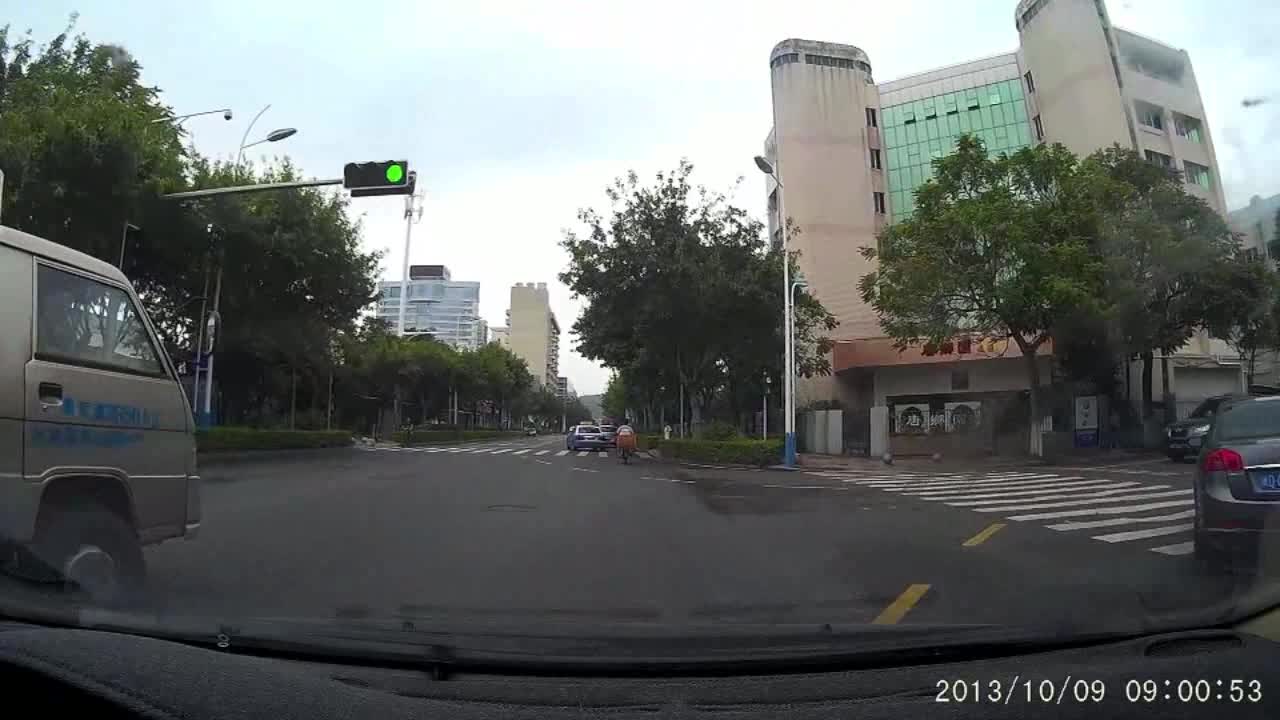This image is a screenshot from dash cam footage taken on October 9th, 2013, at 9:00 AM. The photo captures a busy city intersection with the traffic lights currently green. Several vehicles, including large trucks and a car at the center of the frame, are in motion. The car is navigating a turn through the intersection, either left or right. A central building with distinctive light blue windows stands prominently in the background, flanked by tall green trees that are planted in front of what appears to be a hospital. Large streetlights on tall beams illuminate the area. The scene is bustling with activity, including a distant cyclist pedaling down the road and additional trucks parked further along the street. The urban setting vividly reflects a typical busy morning in the city.